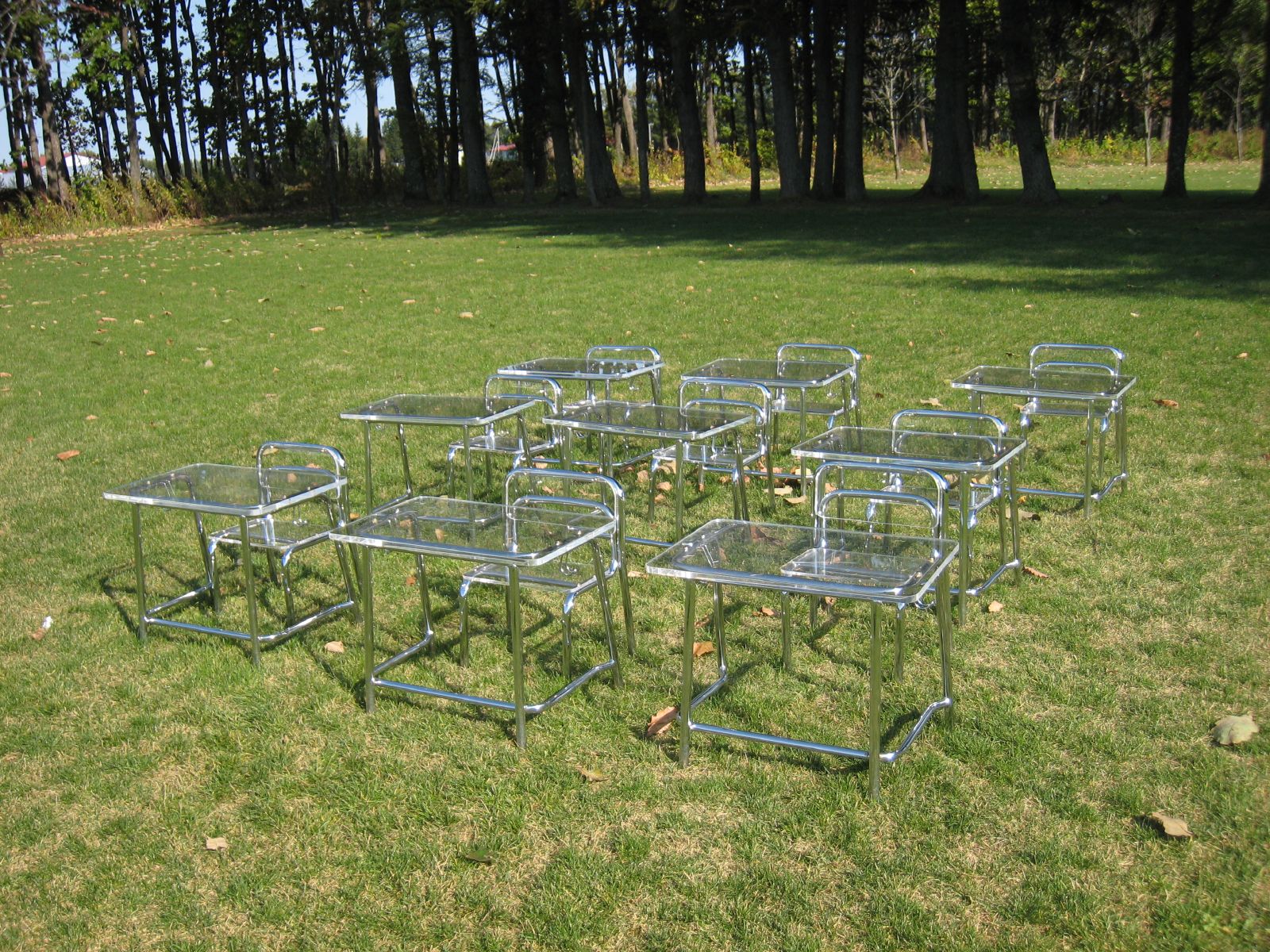The photograph, in vivid color and landscape format, captures a peculiar scene where nine student desks are meticulously arranged in a three-by-three grid, creating a diamond formation when viewed head-on. Each desk sits evenly spaced in the middle of a lush, sunlit grass field. The desks, with their sleek, transparent glass surfaces, reveal the greenery beneath and are supported by metallic, silver legs matching the silver-toned chairs that are attached to them. A distinct line of tall trees serves as a natural barrier, dividing the grassy expanse from another field beyond, under a white sky. Scattered around the desks are a few dead leaves, adding a touch of realism to the otherwise surreal setting.